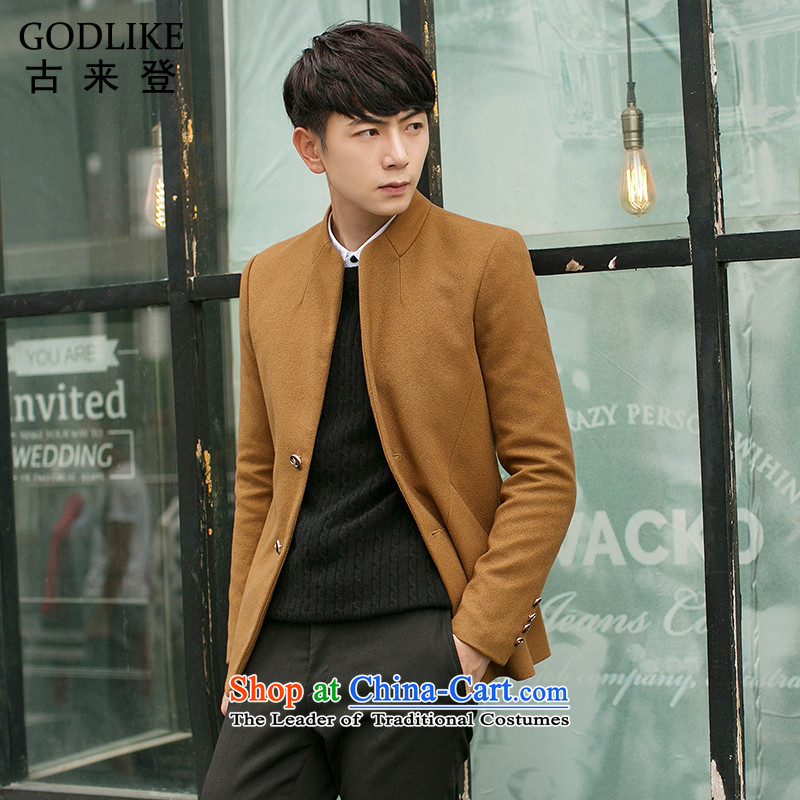A young Asian man, likely around 18 to early 20s, poses as a model in a marketing advertisement. Dressed sharply, he's seen in a brown suede blazer adorned with various gold buttons and black cufflinks, layered over a black sweater and white undershirt, paired with either black or gray dress pants. He gazes seriously over his left shoulder, his left side slightly angled towards the camera, with medium-length black hair and a clean-shaven face. He leans against a rustic building that features worn paint and frosted windows with black trim, with an exposed light bulb hanging inside. Behind him, parts of indistinct lettering on the building include "ACK JEANS CO." In the upper left corner of the image, the word "GODLIKE" appears in bold black capital letters with accompanying Chinese characters below. At the bottom center, the promotional text reads "SHOP AT CHINA-CART.COM" in red, green, and blue letters, followed by the tagline "The Leader of Traditional Costumes" in black serif font. The scene is lit by natural daylight, adding to the authenticity and appeal of the setting.